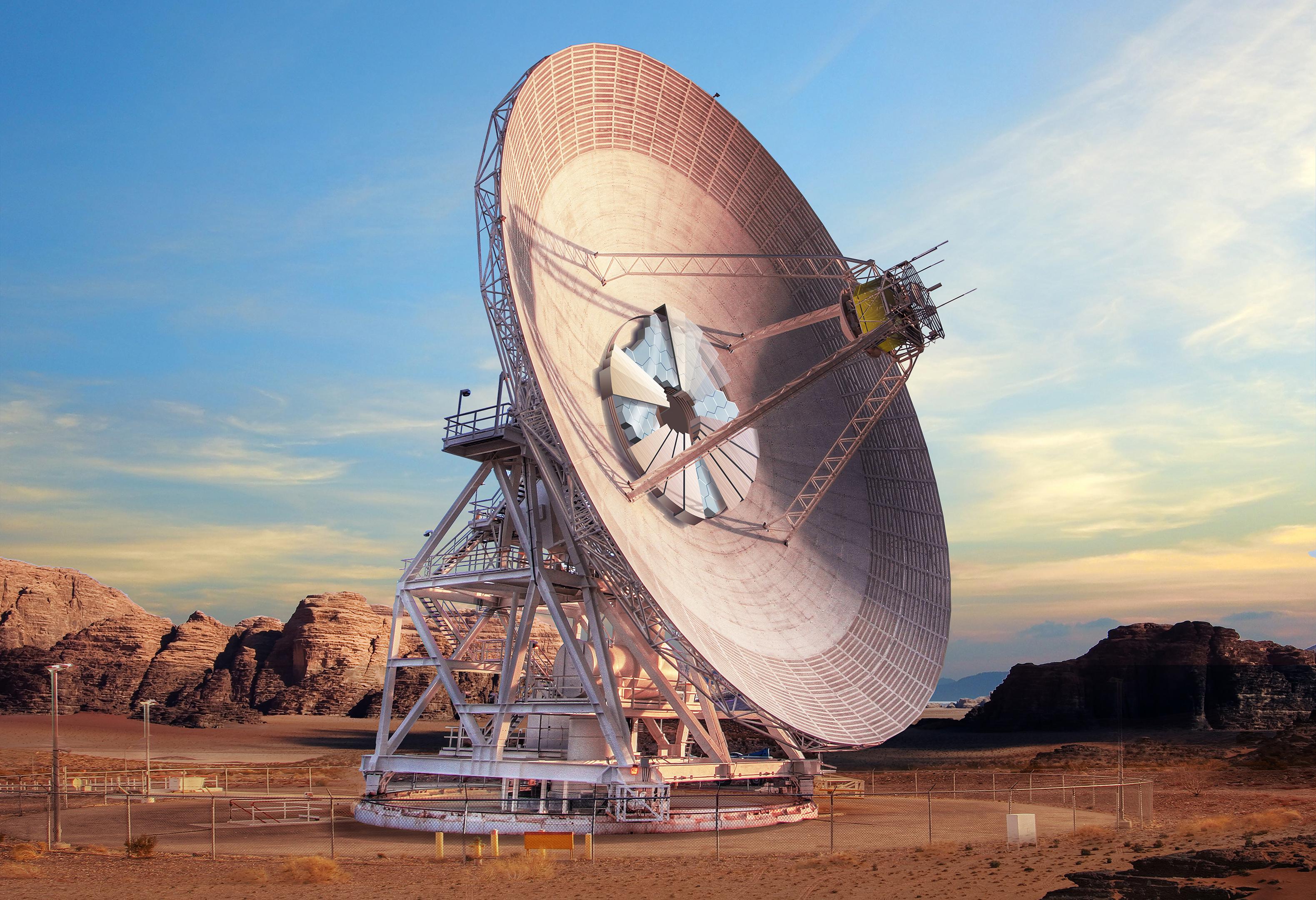The image depicts a vast desert landscape under a clear blue sky with minimal clouds on either side. Dominating the scene is an enormous metal satellite structure, painted white, towering as high as a six-story building. Positioned centrally, the satellite dish is massive, angled towards the right and slightly upwards, giving it an oval appearance. Its dish, constructed with metal panels forming a grid pattern, transitions from light to dark gray and features a concave center.

The center of the dish showcases a complex array of hexagonal, mirror-like objects, partially covered with semi-transparent materials, providing a reflective appearance. Four arm-like structures resembling scaffolding extend from the center, culminating in a pointed antenna or ray, further adding to the intricate design.

The satellite rests on a sturdy, likely rotatable concrete base, surrounded by metal I-beams and brackets, interconnected with numerous bolts and rivets. These components hint at the satellite's ability to pivot on its axis. A metal chain-link fence encircles the satellite, accompanied by several street lights, ensuring security around the installation.

The backdrop features a range of small rocky cliffs to the left and right, composed of sandstone hues varying from dark to light brown, emphasizing the arid environment. Sparse brown leaf shrubs dot the sandy ground, enhancing the desert's barren aesthetic. The entire scene bathes in the golden hue of the setting sun, capturing the expansive, airy feel of this remote, desert location, possibly in regions like Utah or Arizona.